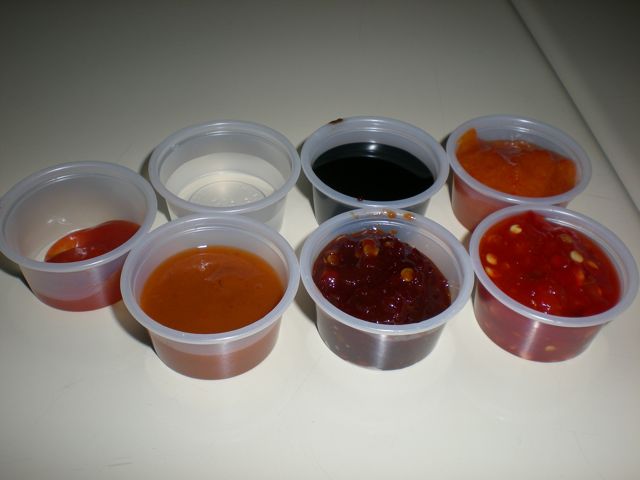On an off-white counter, a detailed photograph showcases seven clear plastic ramekins arranged in two rows. These small condiment cups each contain different sauces, providing a colorful and varied selection. The first ramekin holds a tiny dab of red or orange sauce, possibly ketchup or a spicy chili sauce due to its minimal amount. The second ramekin is three-quarters full of a clear liquid, likely vinegar. The third ramekin contains a brown liquid, filled three-quarters up, possibly soy sauce or teriyaki. The fourth ramekin is nearly full with what appears to be ketchup. Below it, the fifth ramekin contains a three-quarters full serving of a red sauce that could be sweet and sour. The sixth ramekin features a thick, chunky brown sauce, also three-quarters full, which might be a type of chutney or relish. The seventh and final ramekin is full to the rim with a red sauce containing visible seeds, resembling a pepper relish or salsa. The image is subtly vignetted with dim lighting, adding focus to the varied textures and colors of the sauces.